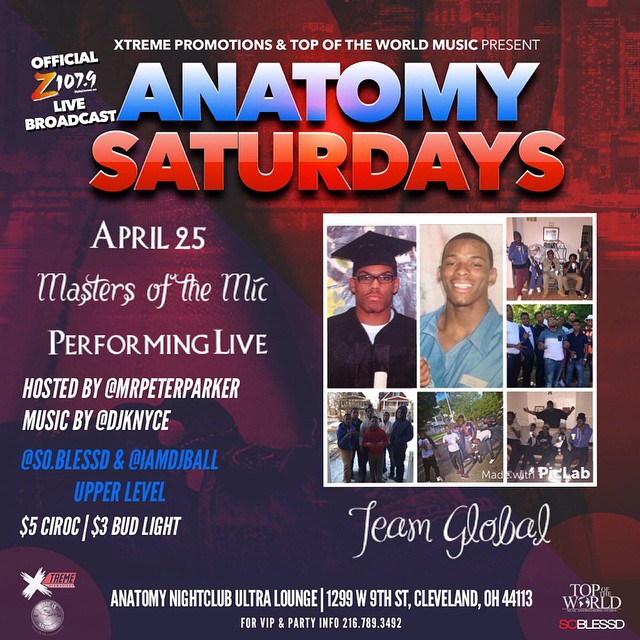The image is an advertisement for an event titled "Anatomy Saturdays," featuring a live broadcast by Z107.9. It prominently highlights "Extreme Promotions and Top of the World Music" as presenters, with the event scheduled for April 25th. The headline act, "Masters of the Mic," is performing live, hosted by Mr. Peter Parker with music by DJ K-NYCE, So Blessed, and I Am DJ Ball. The flyer offers $5 for Cîroc and $3 for Bud Light drinks.

The design includes a collage of images depicting predominantly African-American individuals in various social settings, such as hanging out in living rooms and graduation photos. Notable group names like "Team Global," "Top of the World," and "So Blessed" are included. The event will be held at the Anatomy Nightclub Ultra Lounge, located at 1299 West Ninth Street, Cleveland, Ohio. The flyer’s background is a mix of blue and red colors. For VIP and party details, a contact number is provided: 216.789.3492. Logos for Extreme and Team Global are also featured in the design.